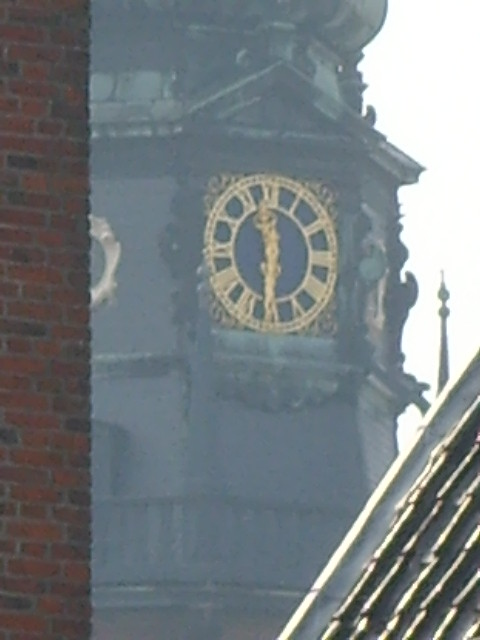This slightly out-of-focus photograph captures a majestic clock tower in an outdoor setting. The clock tower, a tall and wide historical structure, dominates the scene. The photographer appears to have zoomed in considerably, likely with a digital camera, resulting in a grainy image quality that suggests the photo may have been taken years ago. The clock itself features an ornate design with a gold face and intricate gold hour and minute hands. Roman numerals mark the hours, adding to its antique charm. Adjacent to the clock tower, the roof of a nearby building with a steep, tiled pitch can be seen, hinting at traditional architectural styles. To the left of the clock, an old red brick building further enhances the nostalgic atmosphere of the photo. Despite its lack of sharpness, the image evokes a sense of timelessness and historical significance.